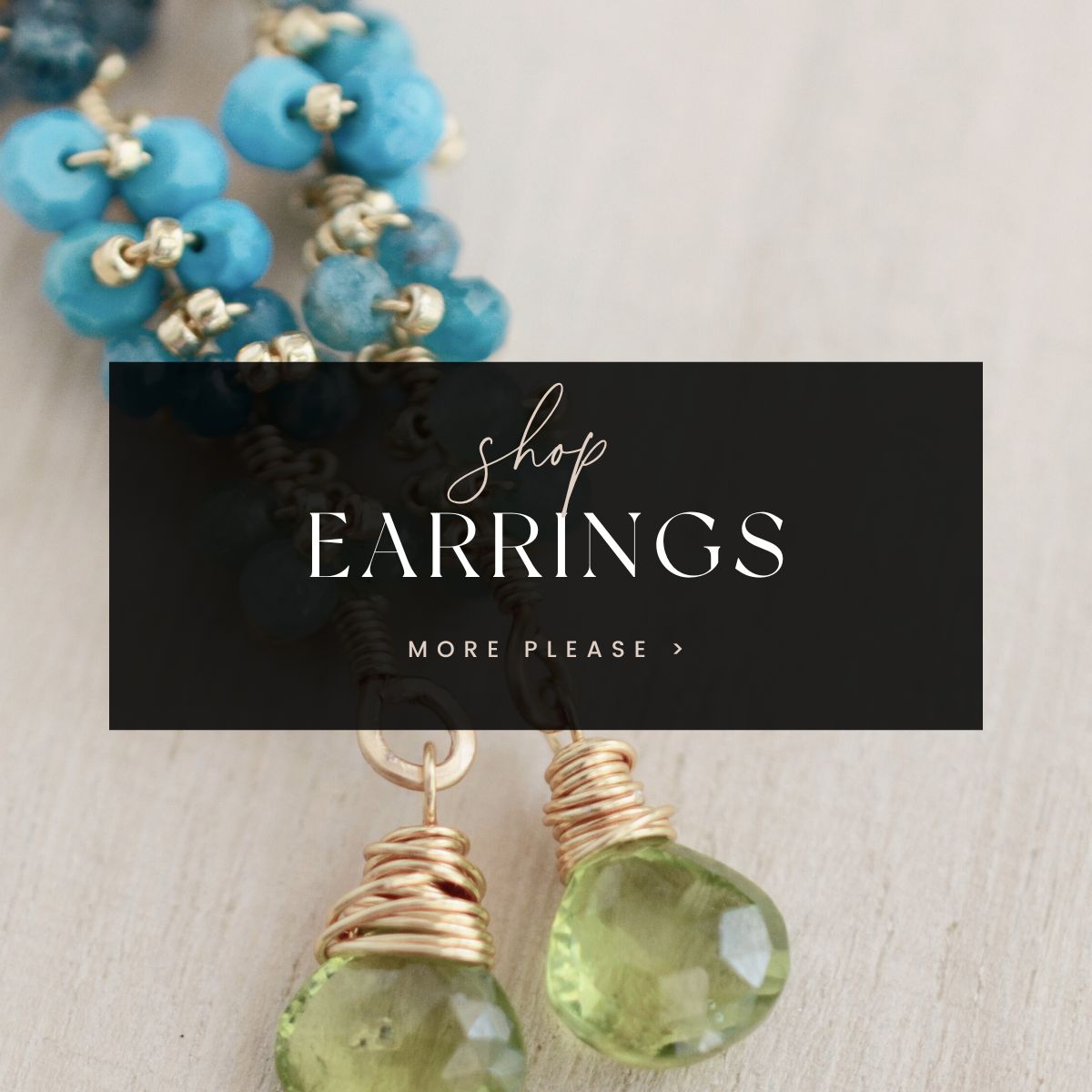The image appears to be a section of a website designed for browsing and shopping jewelry. Dominating the center is a black rectangle with elegant, loopy script that reads "shop" and below it in a bold, clean font, "EARRINGS". Further down, there's an underlined phrase "MORE PLEASE," accompanied by an arrow, suggesting a clickable link for browsing additional earrings.

The background of the image features a light or whitewashed wooden surface on which various pieces of jewelry are displayed. The focal point includes two types of earrings. The first pair, located at the bottom, consists of green amethyst-like gems wrapped in copper wire, accented by small turquoise beads hanging in a chandelier style. Above these, there are silver earrings with blue turquoise beads arranged in a draping formation. Together, these elements seamlessly blend into an engaging and inviting shopping interface for jewelry enthusiasts.